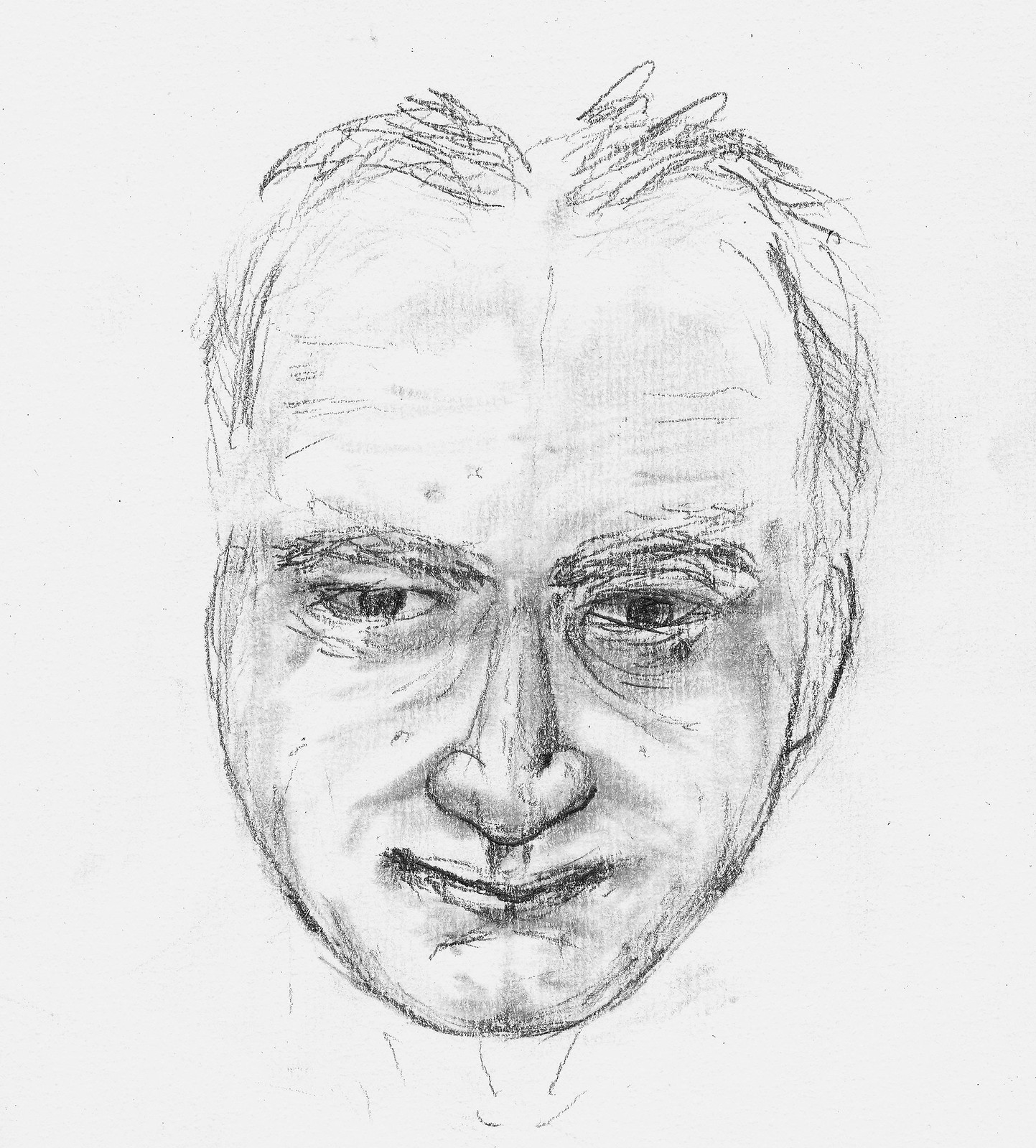This detailed pencil sketch captures a man's face in a striking portrait format, drawn on a square piece of white paper. The face is slightly angled downwards but maintains a full frontal view, gazing directly at the observer with an intense stare. The artist has employed intricate shading techniques, particularly around the nose and eyes, to bring a sense of depth and realism to the sketch. The man's eyebrows are thick and bushy, adding to his stern appearance, while subtle bags under his eyes hint at fatigue or age. His mouth is a straight line, exuding a neutral, almost stoic expression. The hair is short and neatly parted in the center, complementing his high forehead, which features several fine wrinkles on either side of the brow, suggesting contemplation or concern. This portrait masterfully combines detailed shading and expert line work to evoke a captivating and evocative image.